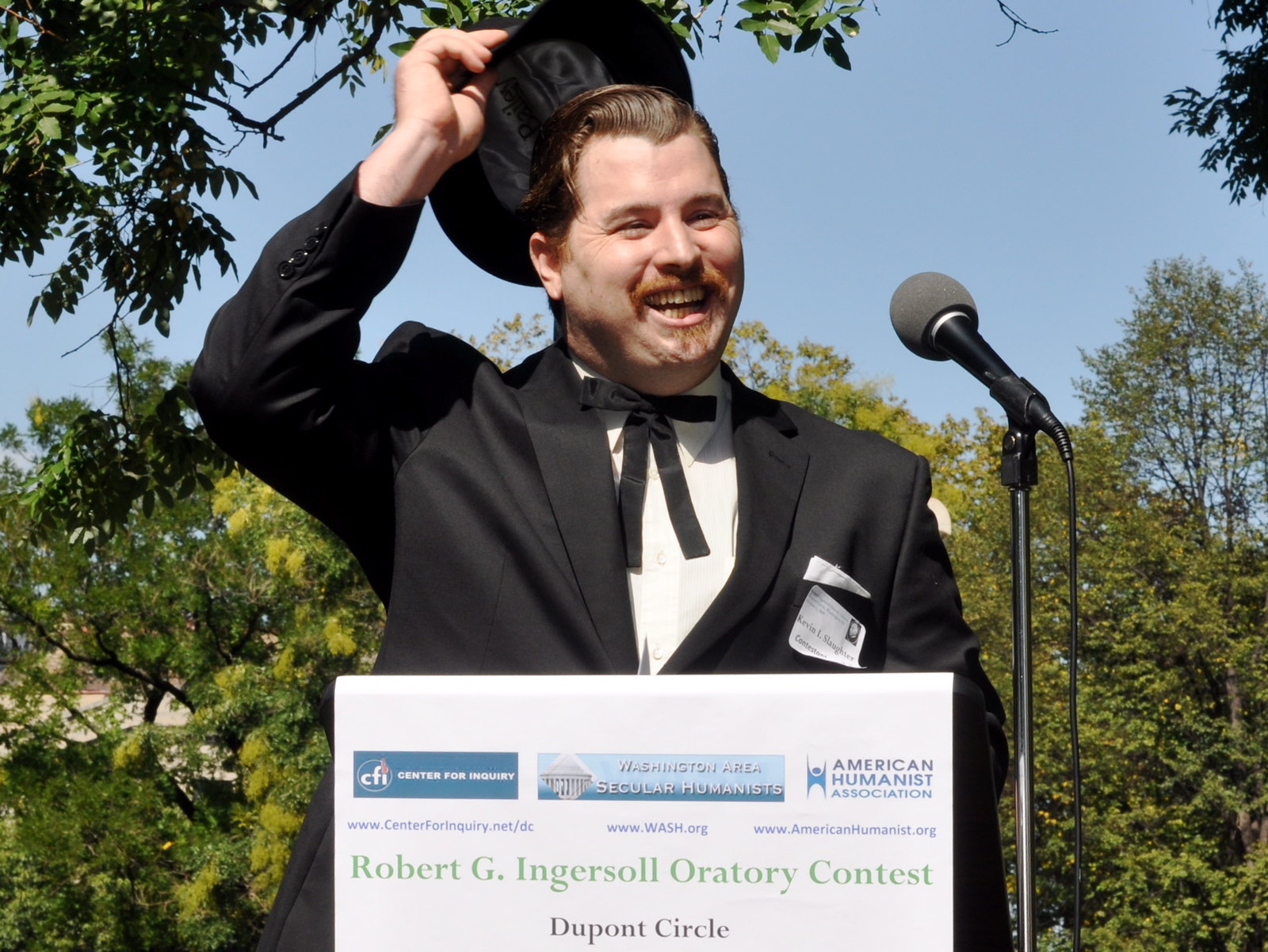In this outdoor photograph, set against a backdrop of abundant trees and a clear blue sky, a man stands at a podium, smiling warmly. He is lifting a black hat off his head with his right hand, revealing his hair. The man is dressed in a black jacket adorned with a white name tag, a white dress shirt, and a black bow tie. He sports a mustache and a small goatee, and speaks into a standing microphone angled towards his face. Below the podium, a white rectangular sign displays “Robert G. Ingersoll Oratory Contest, DuPont Circle,” accompanied by the logos and names of sponsors: CFI (Center for Inquiry), Washington Area Secular Humanists, and the American Humanist Association, along with their respective URLs: www.centerforinquiry.net/dc, www.wash.org, and www.americanhumanist.org.